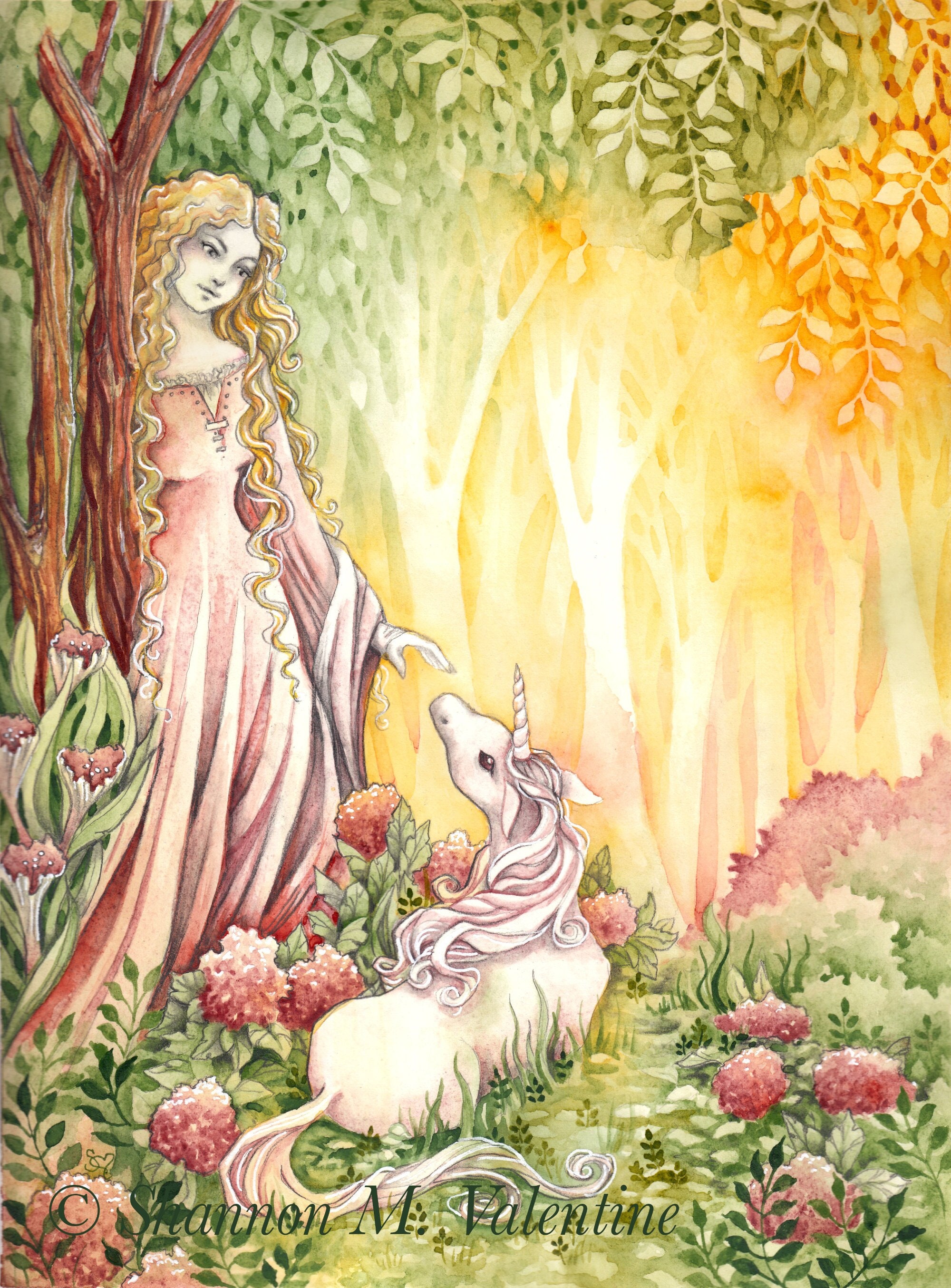This detailed drawing, titled "Shannon M. Valentine," depicts an enchanting outdoor scene featuring a young, white woman in her teens or twenties. The woman, with long, flowing blonde hair parted on either side and cascading almost to her knees, is elegantly dressed in a light pink gown with full sleeves that extend past her feet. She seems to be leaning slightly against a tree amidst a lush setting adorned with flowers and greenery.

In the foreground, the woman is reaching her hand towards a small unicorn that sits or lies on the ground, looking up at her lovingly. The unicorn, primarily white with a light pink mane and a distinctive horn atop its head, is surrounded by large red flowers and green plants.

The backdrop of this picturesque scene is a forest with trees that have a shiny, almost ethereal quality, displaying hues of orange. Overhanging green leaves dominate the top portion of the image, gradually transitioning to orange leaves in the top right-hand corner, perhaps illuminated by sunlight filtering through, adding a magical aura to the forest setting. The grass around the scene is green, and pink flowers embellish the area, enhancing the overall whimsical and fairy-tale-like atmosphere.